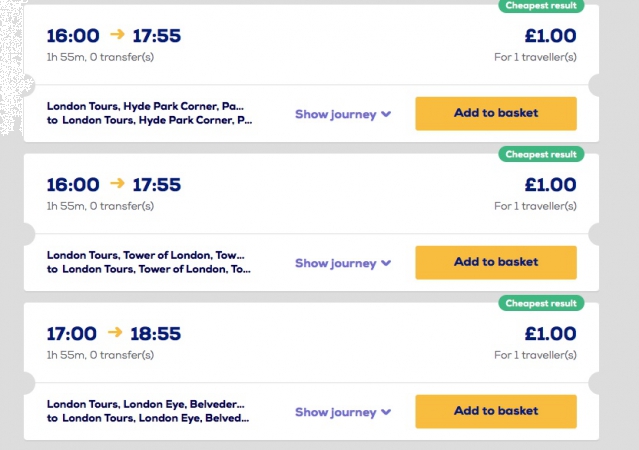This image depicts a page displaying various flight tickets, organized into three distinct sections with white backgrounds. Each section provides detailed information about a specific flight option. 

1. **Top Section:**
   - **Departure Time:** 16:00 
   - **Arrival Time:** 17:55 
   - **Flight Duration:** 1h 55m 
   - **Transfers:** 0 
   - **Price Indicator:** "Cheapest result" highlighted in green 
   - **Price:** £1 listed for one traveler in grey text
   - **Journey Description:** "London Tours Hyde Park Corner PA" (incomplete with dots)
   - **Actions:** Options to "Show Journey" and "Add to Basket" via a yellow button.

2. **Middle Section:**
   - Presents similar details to the top section with respective times and descriptions, presented in a similar format.

3. **Bottom Section:**
   - **Departure Time:** 17:00 
   - **Arrival Time:** 18:55 
   - **Flight Duration:** Also 1h 55m and 0 transfers, similar descriptions and actions available as in the other sections.

Overall, the image is a neatly organized comparison of flight options, clearly highlighting times, prices, and other relevant travel details for easy selection and purchase.